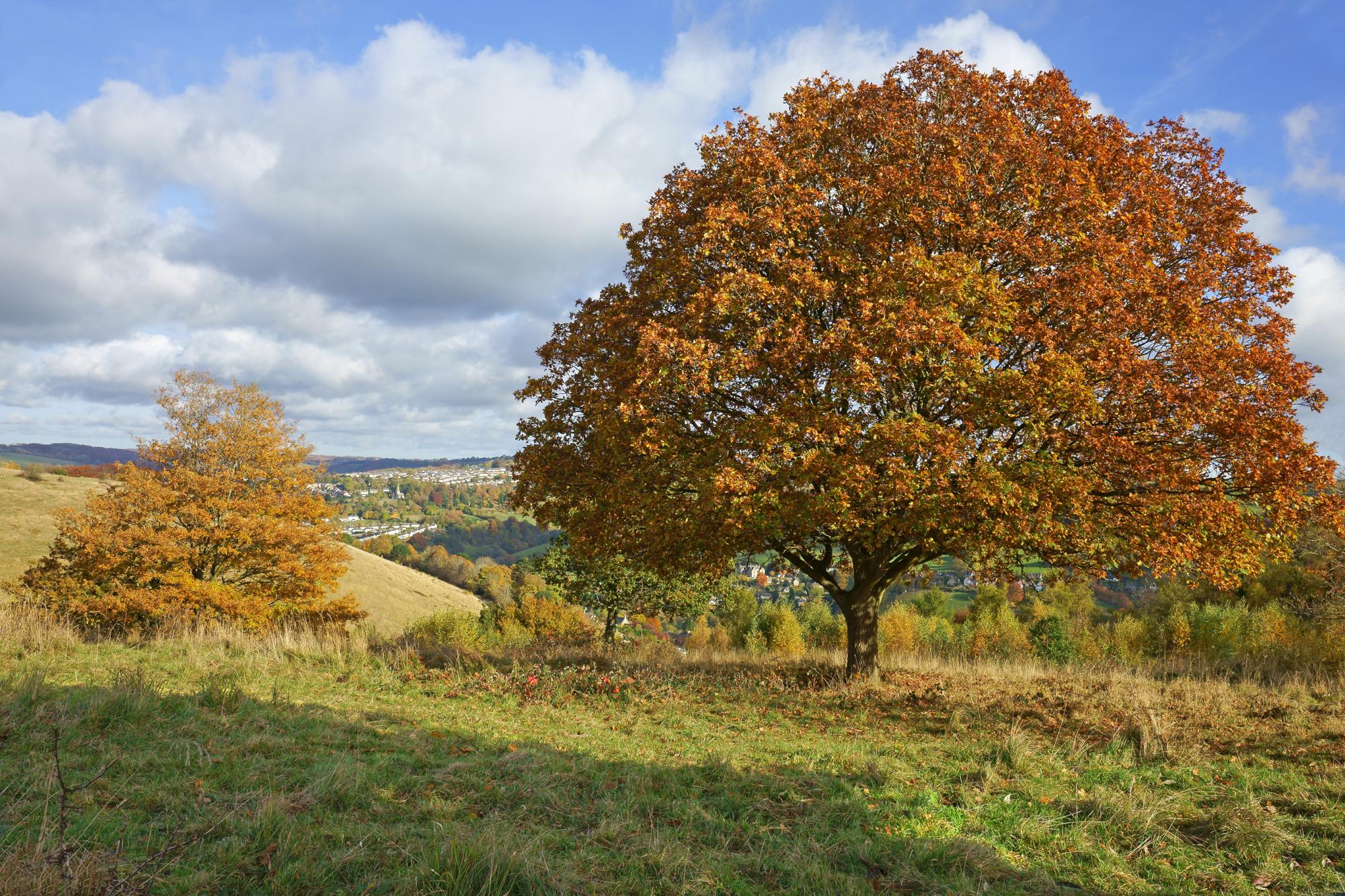This photograph captures a serene fall landscape dominated by a majestic tree positioned towards the right side of the image. The tree displays a stunning array of rust-colored and yellow leaves, with hints of green still visible, signaling the transition of seasons. Standing to the left of the main tree is a smaller tree, its leaves shimmering in golden hues. 

The ground beneath and around the trees is a mixture of green grass interspersed with patches of sun-burnt, browning grass and exposed dirt. This creates a natural, unmanicured look that suggests an untouched, rural setting. 

In the background, rolling hills extend into the horizon, accompanied by a few scattered, white houses that add a quaint touch to the picturesque scene. Above, the sky is a brilliant blue, adorned with fluffy, white cumulonimbus clouds, casting soft shadows on the landscape below. 

The overall composition of the image is devoid of people and text, allowing the viewer to fully absorb the tranquil beauty and natural details of this autumnal setting.